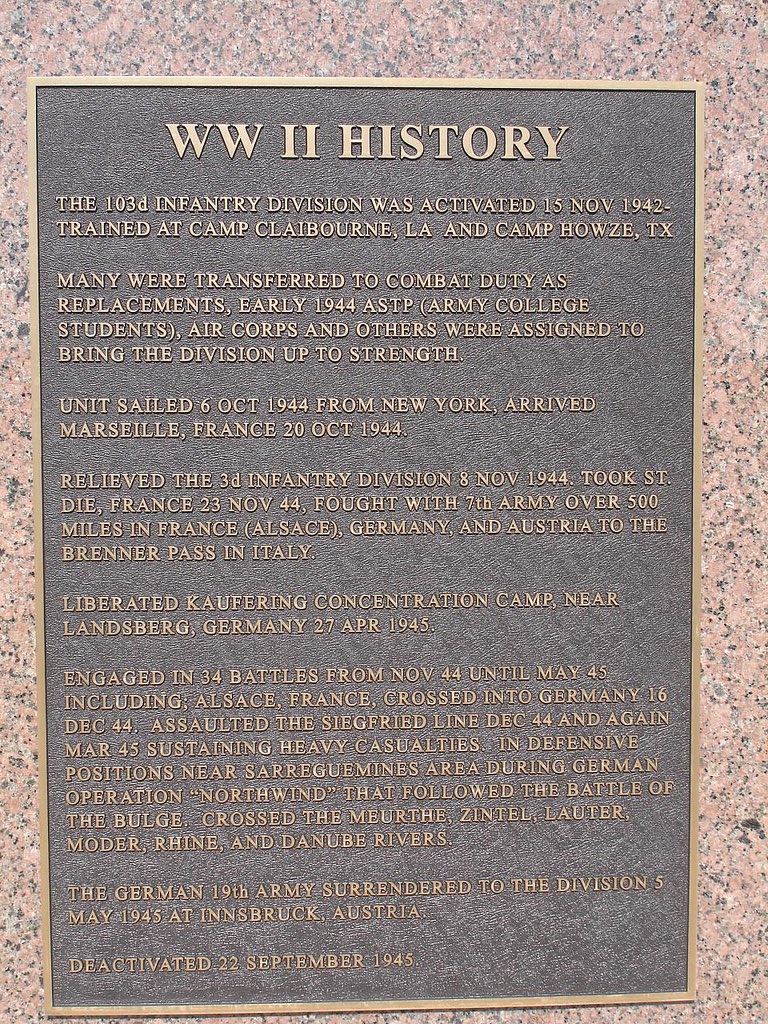This is a detailed photograph of a World War II history plaque dedicated to the 103rd Infantry Division. The plaque is elegantly affixed to a large, speckled stone monument that combines black and orange tones, framed in gold or bronze. The plaque itself has a black background with raised gold lettering and a gold or bronze frame. At the top center, in bold print, it reads "World War II History," followed by a detailed account of the 103rd Infantry Division's service.

The text on the plaque states that the division was activated on November 15, 1942, and trained at Camp Claiborne, Louisiana, and Camp Howze, Texas. Early in 1944, many ASTP Army College students, Air Corps members, and others were assigned to bring the division to full strength. The division sailed from New York on October 6, 1944, arriving in Marseille, France, on October 20, 1944. They relieved the 3rd Infantry Division on November 8, 1944, and captured Saint-Dié, France, on November 23, 1944.

The division fought with the 7th Army over 500 miles across France, Alsace, Germany, and Austria, culminating at the Brenner Pass in Italy. They liberated the Kaufering concentration camp near Landsberg, Germany, on April 27, 1945, and engaged in 34 battles from November 1944 to May 1945, including the Alsace region. They crossed into Germany on December 16, 1944, and assaulted the Siegfried Line in December 1944 and again in March 1945, enduring heavy casualties near Sarreguemines during German Operation Northwind following the Battle of the Bulge. The division also crossed the Meuse, Zintzel, Lauter, Moder, Rhine, and Danube Rivers.

The German 19th Army surrendered to the division on May 5, 1945, at Innsbruck, Austria. The division was deactivated on September 22, 1945.